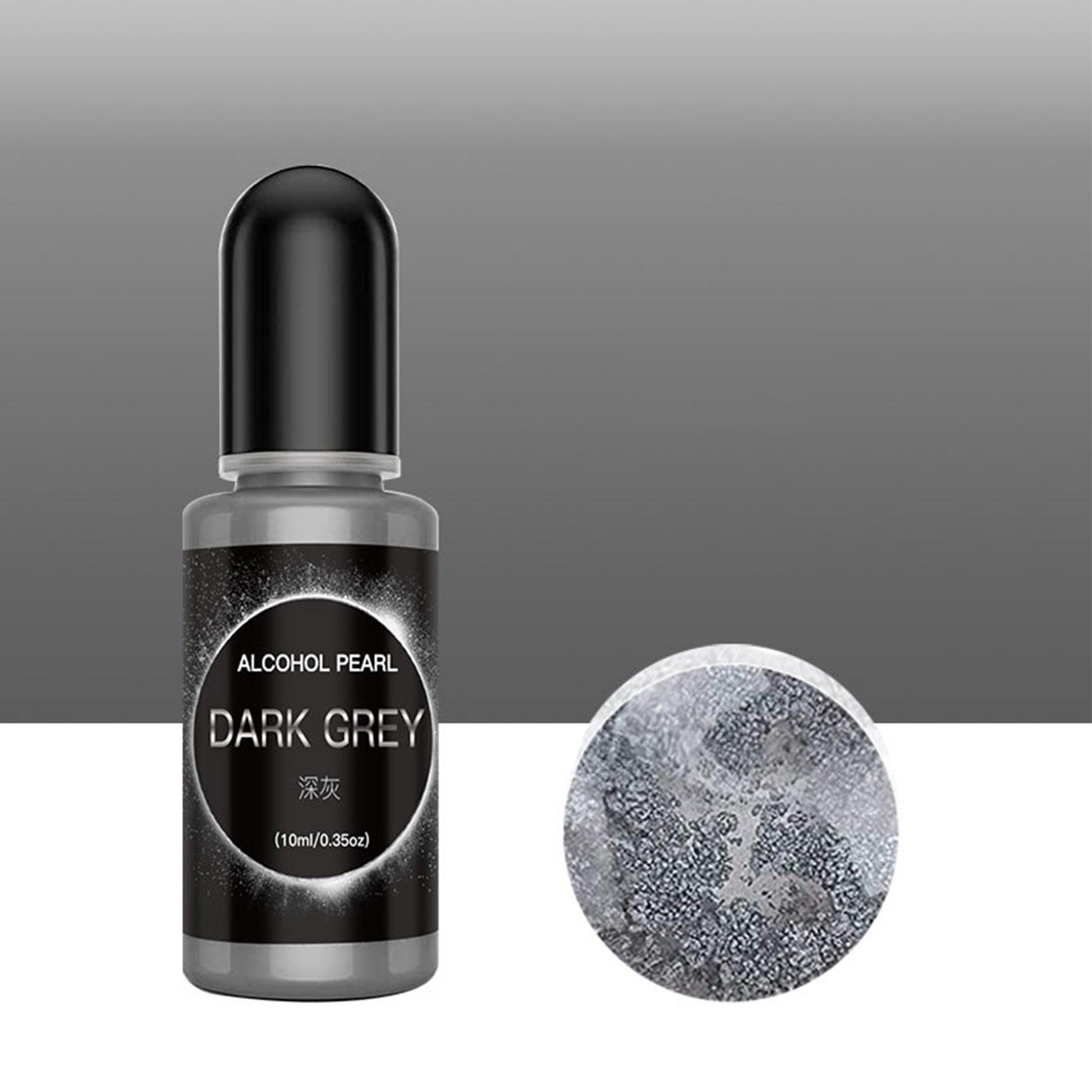The image is a professionally designed black and white advertisement featuring a product on a white and gradient gray background. In the lower section, an elongated rectangle fades from dark gray at the top to light gray at the bottom. On the left side, there’s a small bottle with a tall, rounded black cap and a sleek, silver-gray body. The bottle is wrapped in a black label that features a central black circle outlined in white with the text "Alcohol Pearl" in white font. Below the central text, "Dark Gray" is written in a mix of gray and white letters, followed by two Chinese symbols. Underneath those, it reads "10ml / 0.35oz" in parentheses. 

To the right of the bottle, there is a circular disc that showcases the product’s dark gray finish, consisting of a mix of lighter and darker gray shades with a textured, granite-like appearance. The disc presumably gives a detailed look at the liquid’s effect or finish once applied. The overall gradient background likely serves to accentuate the contrasting elements and colors of the product.